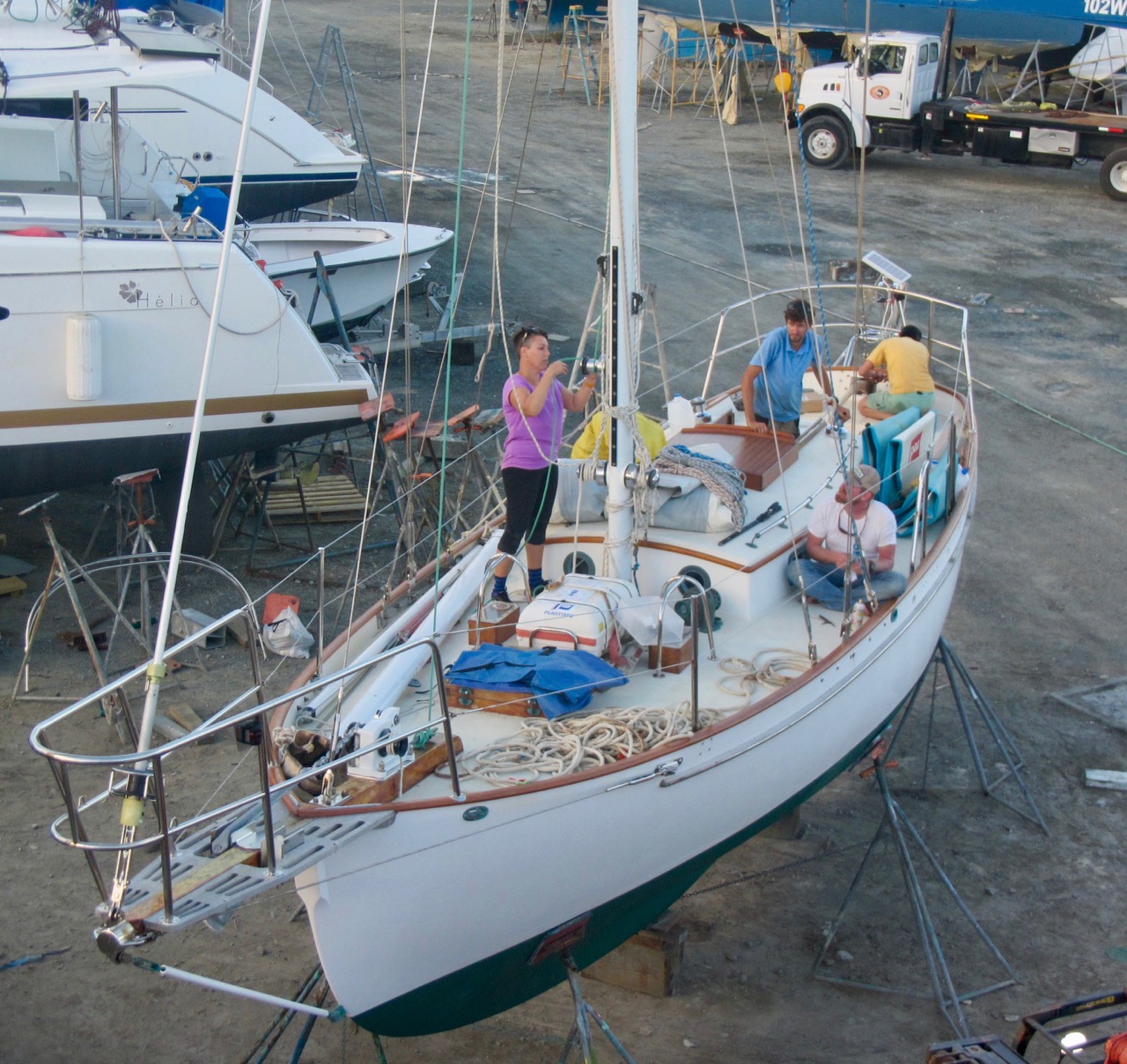This outdoor photograph captures a large parking lot filled with boats propped up on metal stands. Central to the image is a white boat with a black bottom, elevated similarly on stands. A crew of four people is actively working on the boat. At the forefront, a man with lighter skin, dressed in a white short-sleeved t-shirt and blue jeans, is sitting cross-legged on the right side of the boat, engaging with a woman across from him. The woman, characterized by her short hair, wears a light lavender (or purple) short-sleeved shirt, black leggings, and black socks, and appears focused on a task involving the boat's mast. Additionally, two more men are seen further in the background, one bent over, actively contributing to the work. Surrounding this boat, a row of similarly docked boats can be observed, giving a unique sense of this temporary dry dock setting.